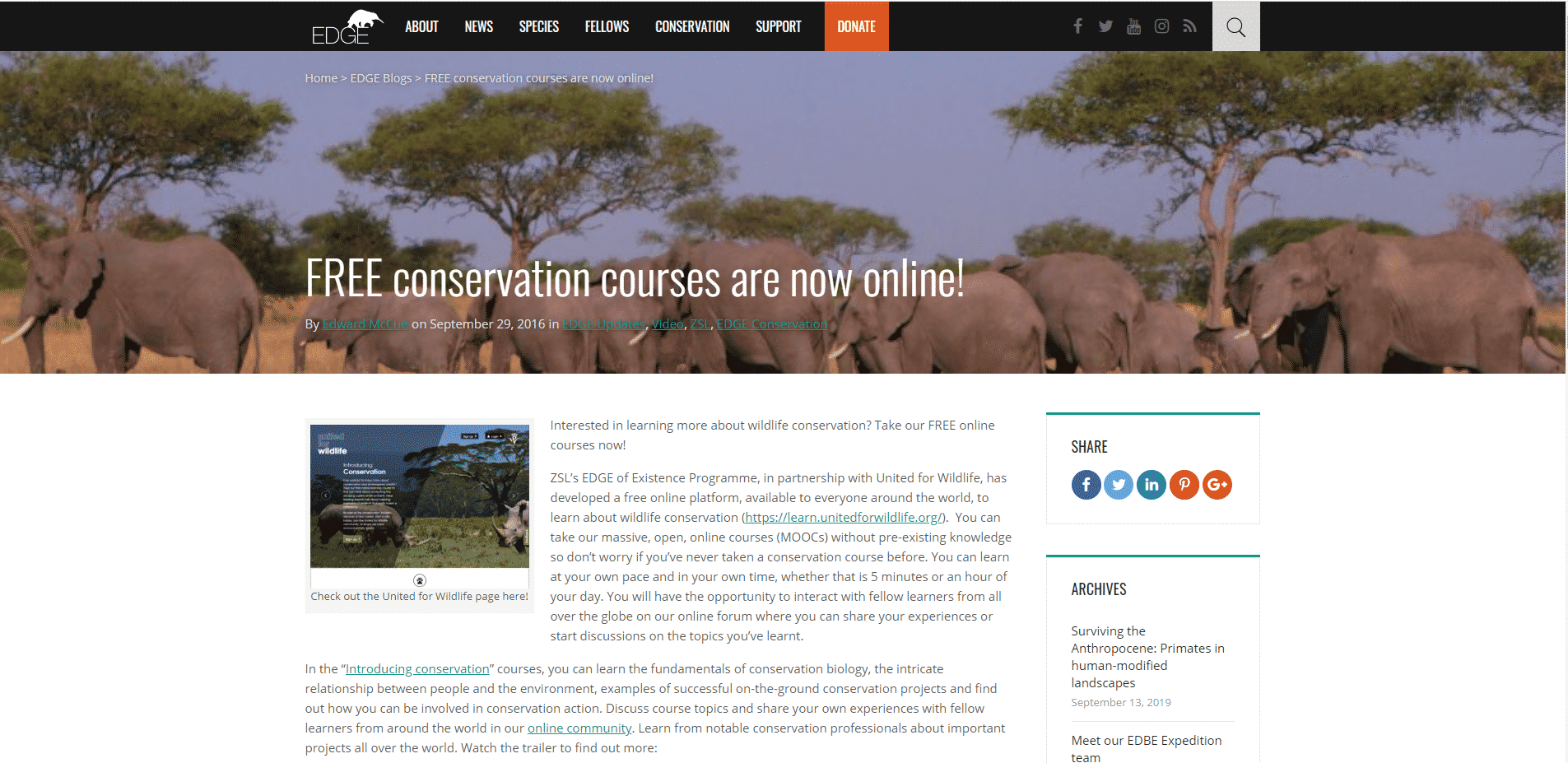The image featured on a conservation course website showcases a well-structured layout aimed at promoting free online conservation courses. At the very top of the screen is a sleek black navigation bar, prominently displaying the company’s logo, "Edge," which features an umbrella-like design over the final letter. The navigation menu includes options such as Home, News, and other items not fully visible in the screenshot.

Beneath the navigation bar, taking up about a quarter of the webpage, is a striking wildlife photograph that serves as the background. This vivid image captures a family of African elephants, varying in size, roaming a brownish grassland with sparse trees typical of the plains. The photograph, which spans the full width of the page, sets a compelling scene for the content.

Overlaying the elephant photo is a bold announcement, "FREE CONSERVATION COURSES ARE NOW ONLINE," with the word "FREE" capitalized to catch the viewer’s attention. Directly beneath this headline, some smaller, centered text is present, although it remains illegible in this screenshot.

The remaining two-thirds of the page is dedicated to additional information presented on a white background with black text. This section includes a justified text layout surrounding another photograph, likely of other wildlife. The content is accompanied by share options featuring recognizable icons for Facebook, Twitter, LinkedIn, Pinterest, and Google, enabling easy sharing across social media platforms. An archives section, presumably containing previous news stories, is also present.

In summary, this detailed webpage effectively combines visual and textual elements to attract interest in free online conservation courses, leveraging striking imagery and clear navigational features.